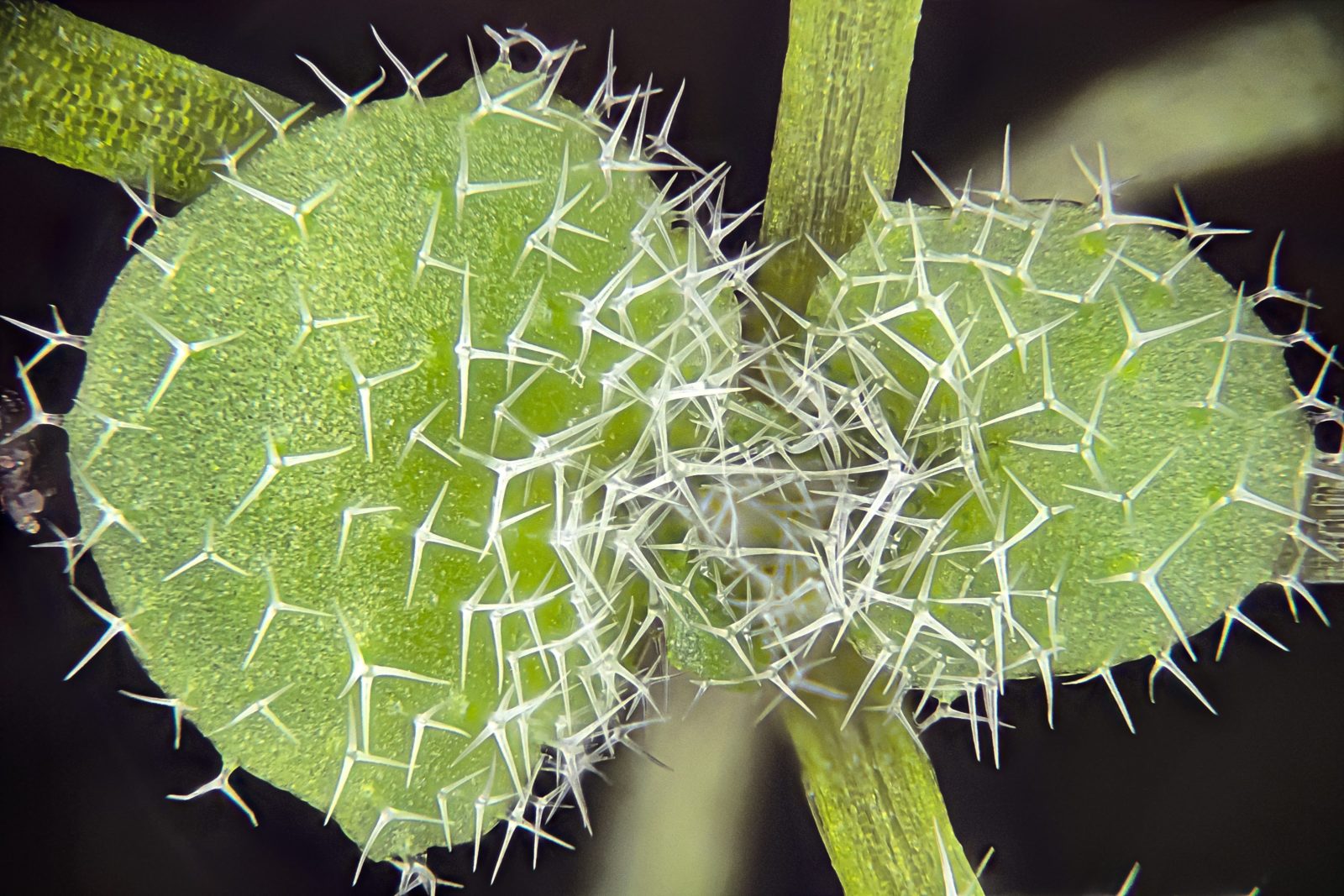The image is a close-up of a round cactus, prominently featuring two large green circles that resemble leaves covered in sharp, white, Y-shaped thorns with three prongs each. These cactus "leaves" are set against a stark black background, which accentuates the details of the plant. In addition to the two main circles, there are noticeable green stripes that look like stems or grass, weaving around and between the circles, some extending across the background and one moving towards the bottom right. The background gradually blurs and fades to black, with hints of additional thorns or spikes visible at the very bottom of the image. The overall composition emphasizes the intricate and somewhat menacing appearance of the cactus, with its distinctive white thorns and deep green coloration.